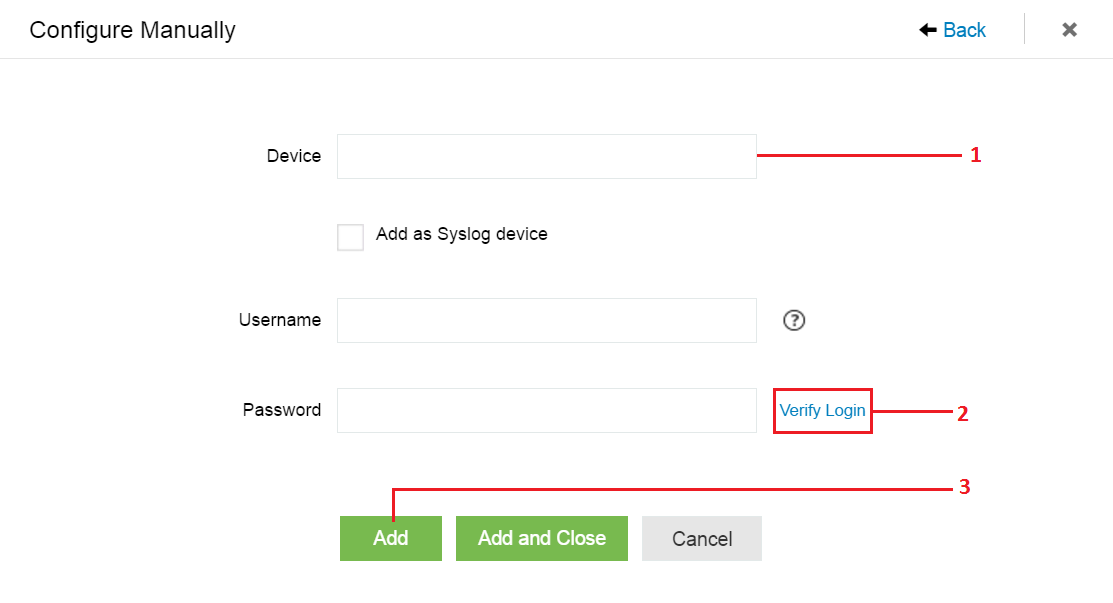The image depicts a fairly minimalistic webpage interface with a white background. Starting from the top left corner, there's a label that reads "Configure Manually." On the far top right, there is a navigation bar that houses a blue back button with a left-pointing arrow, followed by an 'X' icon for closing or canceling the prompt.

Beneath this navigation bar, the main content area begins with a labeled section called "Device." This section includes a text box designed for user input, flanked on the right by a red line marked with the number "1." 

Below this, another line of text reads "Add a Syslog Device", accompanied by a small checkbox to the left for enabling this option. 

Further down, there is a "Username" field with an input box, next to which lies a question mark icon, serving as a help or information button. 

Directly beneath the username field is a "Password" entry section. Adjacent to this, on the right side, is a clickable blue text labeled "Verify Login," enclosed within a red box labeled with the number "2."

At the bottom of the page, there are three action buttons: "Add," "Add and Close," and "Cancel." The "Add" and "Add and Close" buttons are both highlighted in green, suggesting they are the primary actions, while the "Cancel" button appears to reset or close the form.

Overall, the interface appears straightforward and user-friendly with clearly labeled fields and actions.